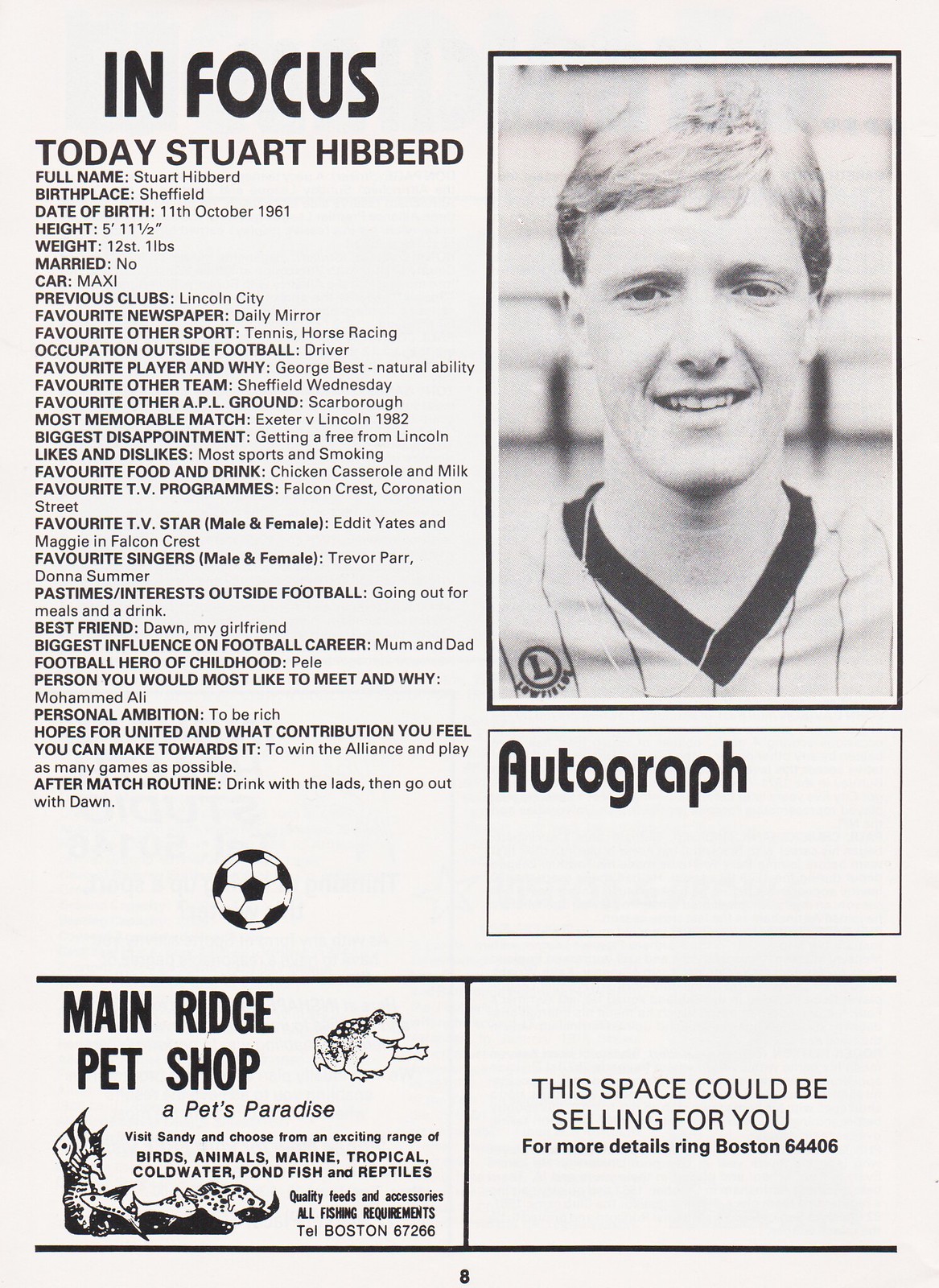The image depicts a nostalgic, black-and-white newspaper page focusing on an individual named Stuart Hibbert. The upper left section prominently features the headline "In Focus Today: Stuart Hibbert," followed by a detailed list of his personal and professional statistics. These include his full name, birthplace (Sheffield), date of birth (11th October 1961), height (5'11 and a half), weight (12st 1lb), marital status (unmarried), car (Moxie), and previous clubs (Lincoln City). The list also covers a wide array of personal preferences and experiences, including his favorite newspaper, other sports, occupation outside football, favorite players, sports teams, hobbies, and more, painting a comprehensive picture of his life and career.

On the right side, there is a headshot of Stuard Hibbert. He's a young, smiling white man with dark blonde or light brown short hair, clad in what seems to be a baseball player's shirt, although only his face and part of his neckline are visible. Below his photo, a box marked "Autograph" appears, but it remains empty.

Beneath Hibbert's detailed profile, the page features two separate advertisements. The first, on the left side, promotes Main Ridge Pet Shop, complete with small drawings of a frog and fish and additional business details. The second ad space to the right remains blank, aside from the text, "This space could be selling for you. For more details, ring Boston 64406."